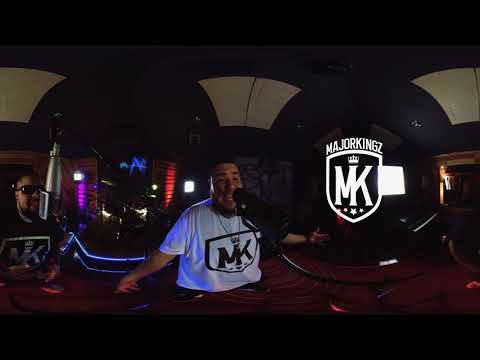In this vivid, color landscape photograph, the central subject is a dark-skinned man, approximately 40 years old, with black hair. He stands at a microphone, singing passionately, with his arms outstretched and eyes focused ahead. He wears a white t-shirt emblazoned with a black "MK" logo encased in a shield shape. This logo is mirrored by another man to his left, who sports black sunglasses and a matching black t-shirt featuring the same "MK" logo, but in white. The scene appears to be indoors, possibly a recording studio, illuminated by an array of colorful lights in purple, blue, and red hues, complemented by regular white lights. The backdrop behind the man to the right forms a fisheye panoramic effect, blending two distinct images: an exterior street view at night with vibrant neon lights and the bold "MAJOR KINGS" text in white, adorned with a crown above it. Both men are holding microphones—silver for the one in the black t-shirt and black for the one in the white t-shirt. A maroon object lies in front of them, while dual-toned black and white patterns decorate the ceiling of the studio, enhancing the dynamic and atmospheric setting.